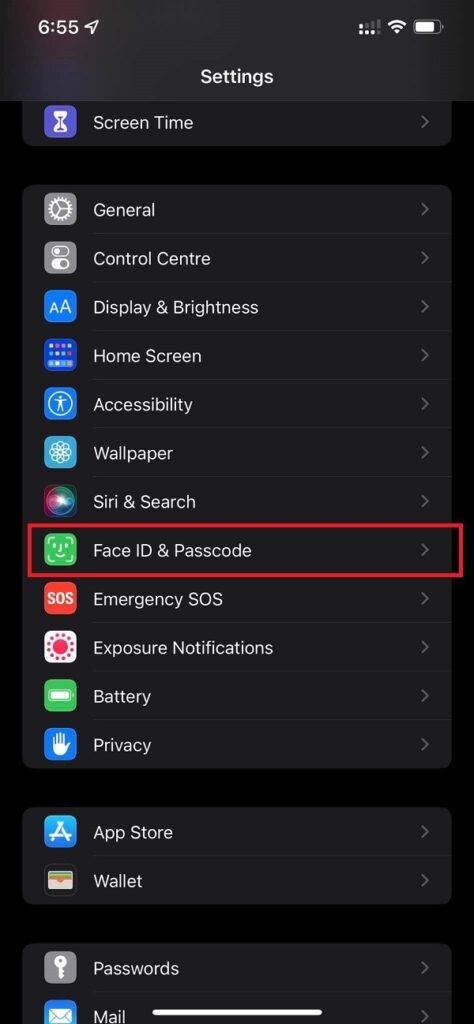The image is a screenshot of a settings menu, featuring a black background with predominantly white and gray text. It is time-stamped at 6:55, as indicated at the top of the screen along with a paper airplane-like icon, a Wi-Fi icon showing one bar of signal strength, and a battery icon. 

The header "Settings" is prominently displayed, beneath which several menu options are arranged in square, clickable boxes, each adorned with specific icons and down arrows for expandable options.

1. **Screen Time**: Represented by a purple and white hourglass icon.
2. **General**: Displayed with a gray and white cogwheel.
3. **Control Center**: Marked by a gray square featuring white icons.
4. **Display & Brightness**: Illustrated by a blue box with two white A's.
5. **Home Screen**: Indicated by a blue box with various colored icons.
6. **Accessibility**: Shown with a blue box and a white cartoonish person icon.
7. **Wallpaper**: Symbolized by a baby blue box with a white flower.
8. **Siri & Search**: Recognized by a multicolored icon consisting of pink, green, and blue elements.

The highlighted section:
- **Face ID & Passcode**: This box is highlighted in red, featuring a green square with a white smiley face.

9. **Emergency SOS**: Depicted by a red square with white "SOS" text.
10. **Exposure Notifications**: Represented by a white box with a pink sun-like icon.
11. **Battery**: Illustrated by a green square with a white battery icon.
12. **Privacy**: Shown with a blue box and a white hand icon.
13. **App Store**: Depicted by a blue background with a white "A".
14. **Wallet**: Illustrated with an olive, white, and brown wallet icon.
15. **Passwords**: Indicated by a gray square with a white key.
16. **Mail**: Represented by a blue square with a white envelope.

The layout concludes with a white line visible at the bottom of the screen, delineating the different sections of the settings menu.